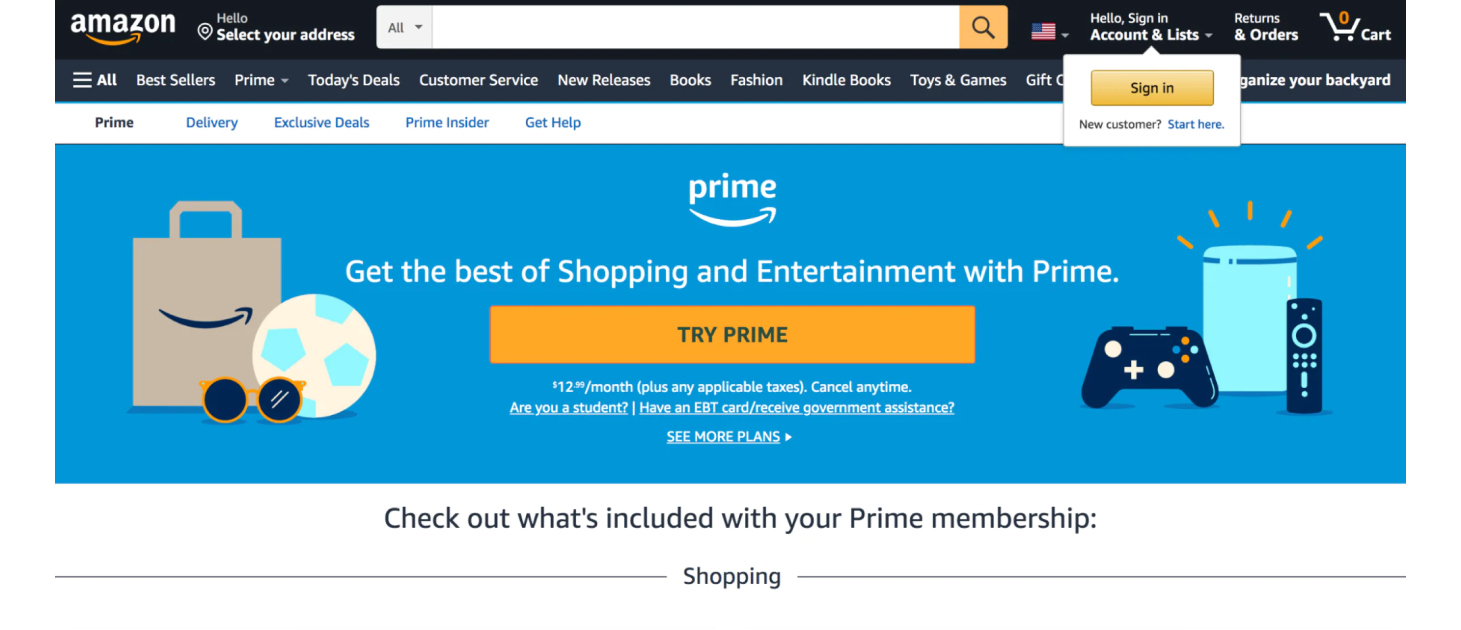**Detailed Caption for Image of Amazon Shopping Website on a Laptop/Computer Screen**

The image is a snapshot of an Amazon shopping website displayed on a landscape-oriented laptop or computer monitor. The lower half of the image is a blank, white background, but the upper section features the familiar black navigation bar seen at the top of Amazon's shopping pages.

**Navigation Bar Details:**

- **Top Black Bar:**
  - **Center:**
    - A notable white search bar stands prominently in the middle. It features an orange square containing a black magnifying glass icon on the right side, and the word "All" in gray letters on the left, indicating the option to search across all categories. A drop-down arrow accompanies the word "All," allowing users to narrow their search categories.
  - **Left Side:**
    - The word "Amazon" is displayed along with the iconic smiley arrow logo.
    - A location icon resembling an inverted teardrop, labeled with "select your address," is also visible.
  - **Right Side:**
    - A US flag icon with a drop-down arrow, providing options for users not shopping in the US.
    - A "Hello, Sign in" section with a pop-up overlay offering links to "Account & Lists" and a yellow "Sign in" rectangle. Below this is a link for new customers labeled "Start here" in blue.
    - A clickable link for "Returns & Orders."
    - A shopping cart icon labeled "Cart" with an orange "0," indicating an empty cart.

**Secondary Blue Bar Beneath the Navigation Bar:**

- **From Left to Right:**
  - A triple-stacked line menu icon next to the word "All."
  - Links for "Best Sellers," "Prime" with a drop-down arrow, "Today's Deals," "Customer Service," "New Releases," "Books," "Fashion," "Kindle Books," "Toys & Games," "Gift Cards" (partially obscured by the Sign-In pop-up), and "Organize Your Backyard."

**Content Below the Bars:**

- **White Space Section:**
  - The word "Prime" in black letters on the left.
  - Four blue clickable links: "Delivery," "Exclusive Deals," "Prime Insider," and "Get Help."

**Large Blue Rectangle Section:**

- **Illustrations:**
  - Left Side: 
    - A gray shopping bag with the Amazon smiley arrow.
    - A white and blue soccer ball and orange-framed sunglasses on the ground.
  - Right Side: 
    - A blue cylinder with orange vertical lines, likely representing an Alexa Echo device.
    - A black game controller and black remote control.

**Text and Buttons:**

- **Center Text in White:**
  - The word "Prime" with the smiley arrow logo below.
  - The phrase "Get the best of shopping and entertainment with Prime."
  - A large orange clickable button saying "TRY PRIME" in all-capital black letters.
  - Small white text below explaining the monthly cost ($12-something) plus applicable taxes, with options to cancel anytime.
  - Underlined clickable links for students and those with an EBT card or receiving government assistance.
  - A link in all caps, "SEE MORE PLANS," with a right arrow, suggesting additional details are available.

- **Bottom Text:**
  - "Check out what's included with your Prime membership."
  - The section title "Shopping."

The description carefully captures the content, layout, and visual details of the image, providing a comprehensive understanding of its elements.